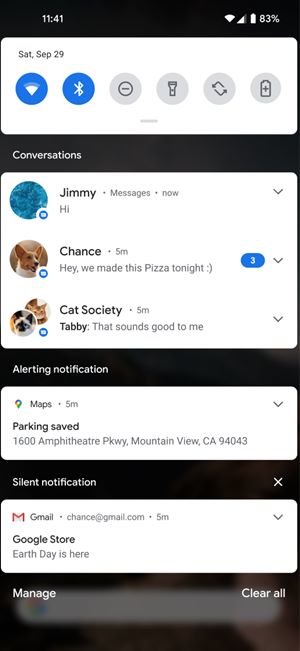The image displays a smartphone screenshot with the notification bar swiped down, revealing a detailed view of various notifications. At the top, the notification bar showcases six icons, indicating active Wi-Fi and Bluetooth connections, while other icons remain inactive. Below this, a series of conversation snippets appear: Jimmy messages with a simple “hi,” Chance shares, “hey, we made this pizza tonight,” and in a group chat named Cat Society, Tabby responds, “that sounds good to me.” Further down, an alerting notification from Maps informs the user of a saved parking location at a specific address. Lastly, a silent notification from Gmail (chance@gmail.com) announces, “Google Store Earth Day is here.” The background of the screen is slightly blurred, keeping the focus on the notifications and active icons.